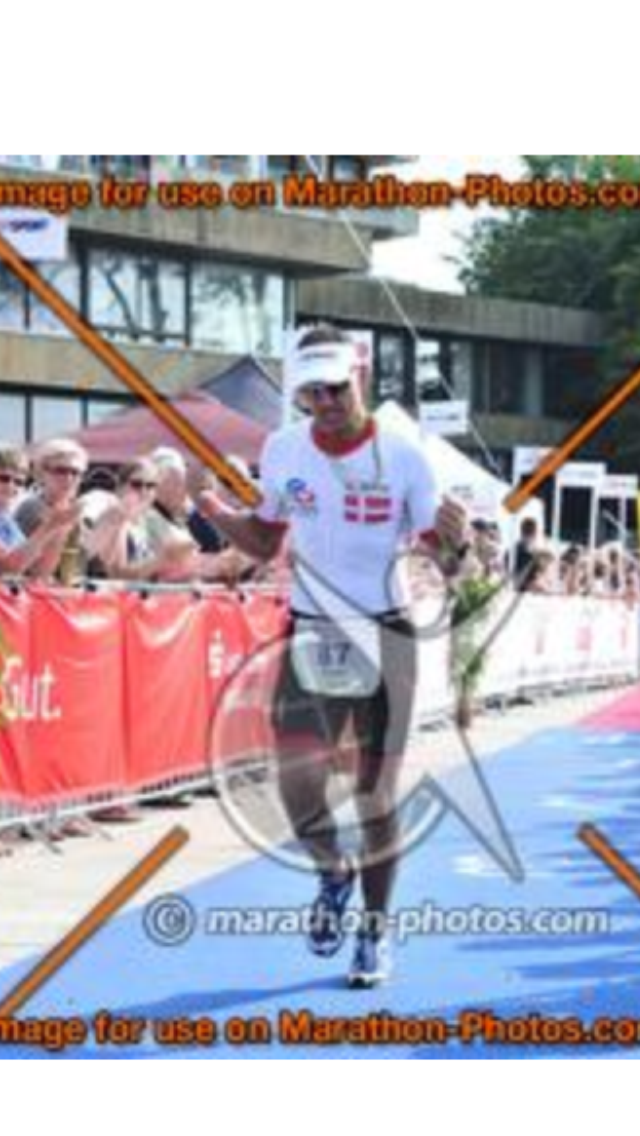The image captures a male participant competing in a race, running on a blue-colored track with orange writing underneath. The athlete is dressed in a white t-shirt with text on it, black pants, blue shoes, and a white cap with an open top. He is in mid-stride with his arms pumping beside him. Behind the runner, there are numerous spectators standing behind a fence. Many of them appear to be older individuals wearing sunglasses. Beyond the spectators, there is a modern-style building with multiple floors and large reflective windows, possibly a grandstand. A tree is also visible in the background. At the top and bottom of the image, there's text that reads, "Image for use on marathon-photos.com," with a watermark logo in the center with the same website text. The overall composition includes some superimposed images giving it a layered effect.